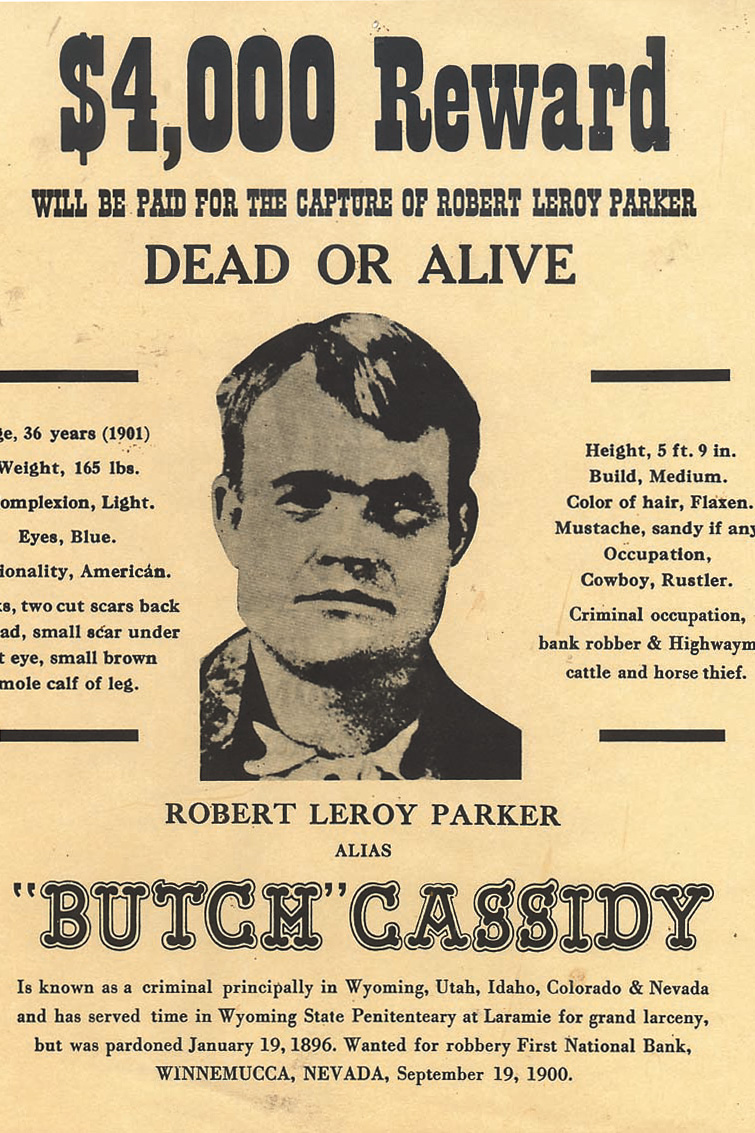The image presents a wanted poster reminiscent of the late 19th or early 20th century, printed on a yellowish-white background. Prominently featured at the top is an offer of a "$4,000 reward for the capture of Robert Leroy Parker, alias Butch Cassidy, dead or alive." Beneath this, a black-and-white photograph of Robert Leroy Parker provides a visual reference, although it's noted to be somewhat rough and unclear. Flanking the photograph are detailed physical descriptions: age 36 (in 1901), 165 pounds, light complexion, blue eyes, American nationality, with distinguishing marks including two cut scars on his back and a small scar under his right eye, as well as a small brown mole on his calf. The poster also outlines Parker’s criminal history, listing offenses like bank robbery, highway robbery, and cattle theft, and indicates his areas of operation as Wyoming, Utah, Idaho, Colorado, and Nevada. The overall impression is of an old-fashioned wanted poster, complete with period-specific typography and layout.